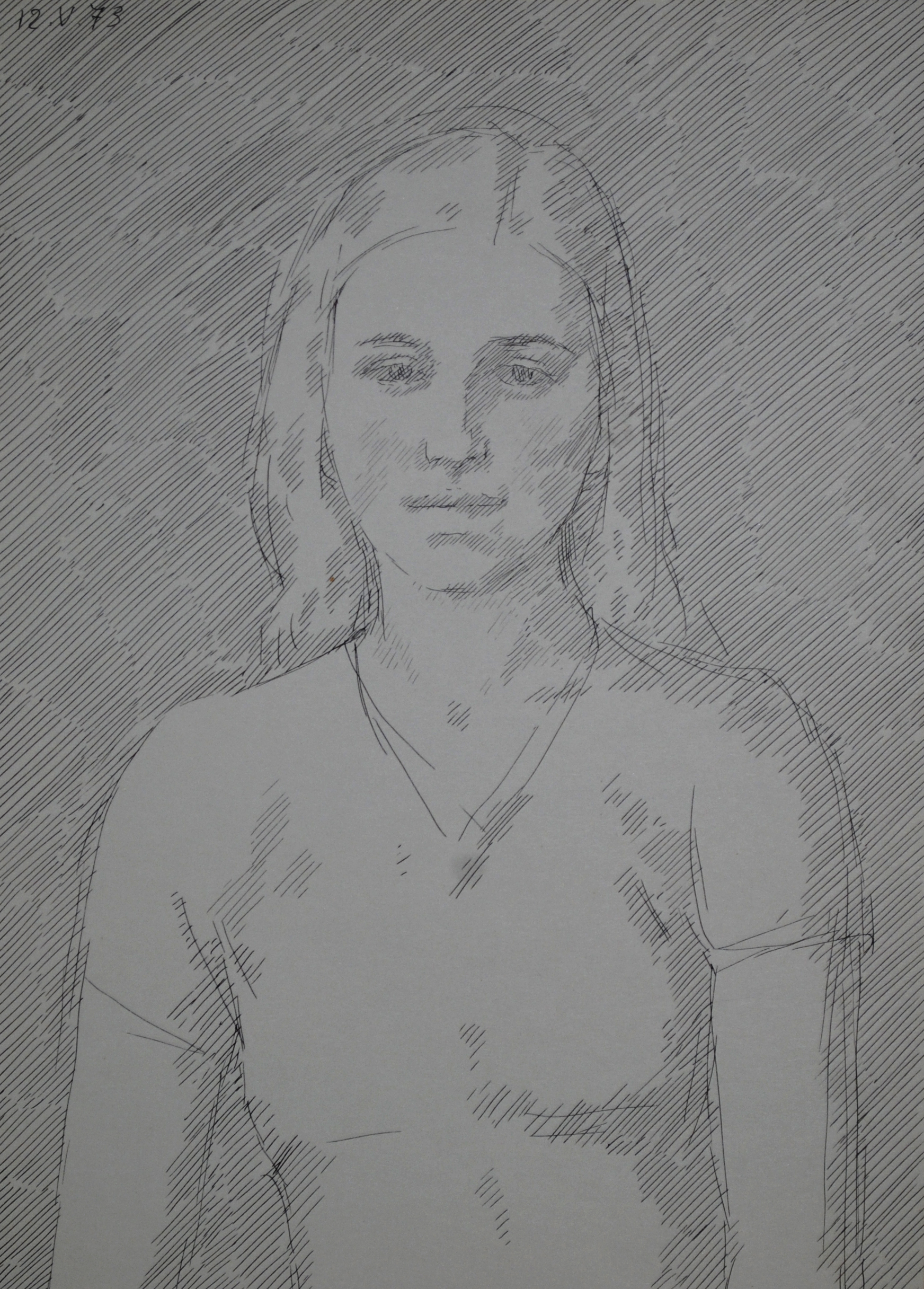This detailed pencil sketch features a young woman in the center, looking slightly to the left with a vacant, somber expression. Her long, straight hair is parted to the right and flows behind her shoulders, obscuring her ears. She has thin black eyebrows, a small nose, and closed lips. The woman is dressed in a V-neck short-sleeved T-shirt, with her bare arms hanging down by her sides, though her hands are not visible. The background consists of dense, diagonal black lines running from the top right to the bottom left, creating a wall-like texture. The entire image is rendered in black and white, capturing a sense of heaviness and introspection in her gaze.